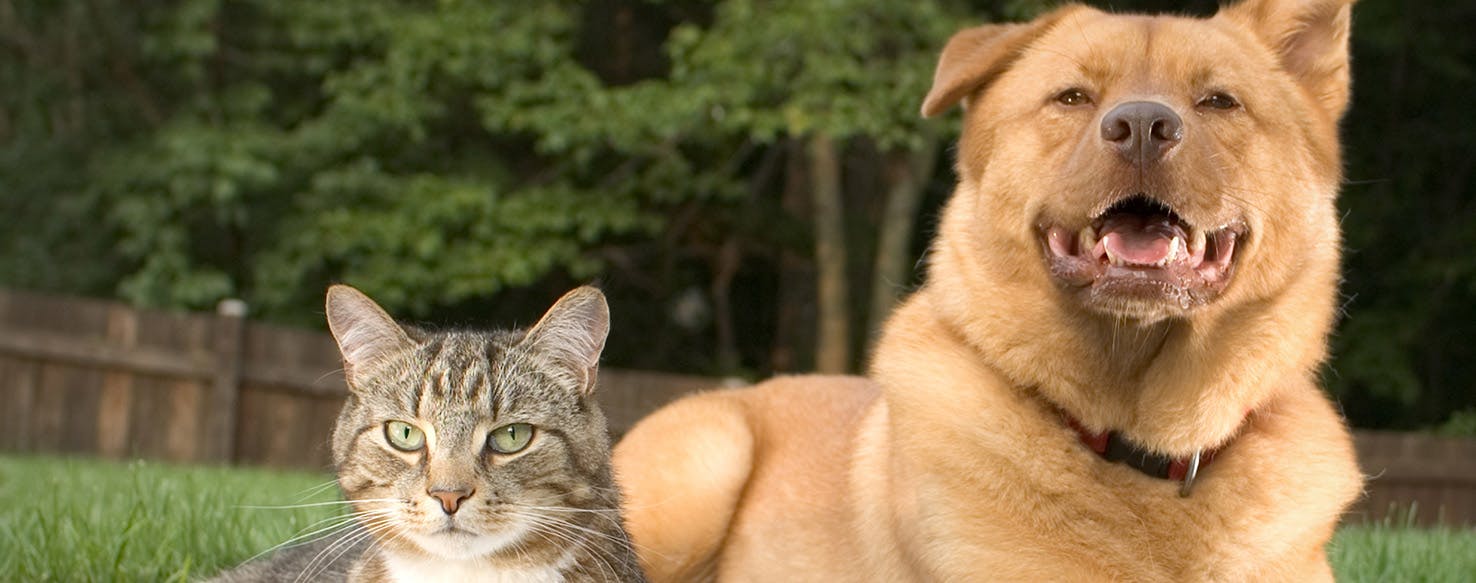In this charming and detailed photograph, a gray tabby cat and a fluffy tan-reddish dog are lying side by side on the grass in a backyard. The cat, positioned on the left, is a grayish color with black stripes, striking green eyes, long whiskers, and a pink nose. It gazes directly at the camera with an expressionless face. The dog, larger and situated on the right, sports a red collar with a silver buckle. This cheerful dog has its mouth open in a pant, revealing a light smile, and its dark brown eyes and black nose stand out prominently. One of its ear flaps rests down, while the other ear listens attentively. Together, they are set against a backdrop of a slightly blurry wooden fence and dense trees, hinting at natural surroundings illuminated by artificial light. Despite the potential suggestion of a superimposed image, the scene captures an endearing moment of these seemingly good buddies.